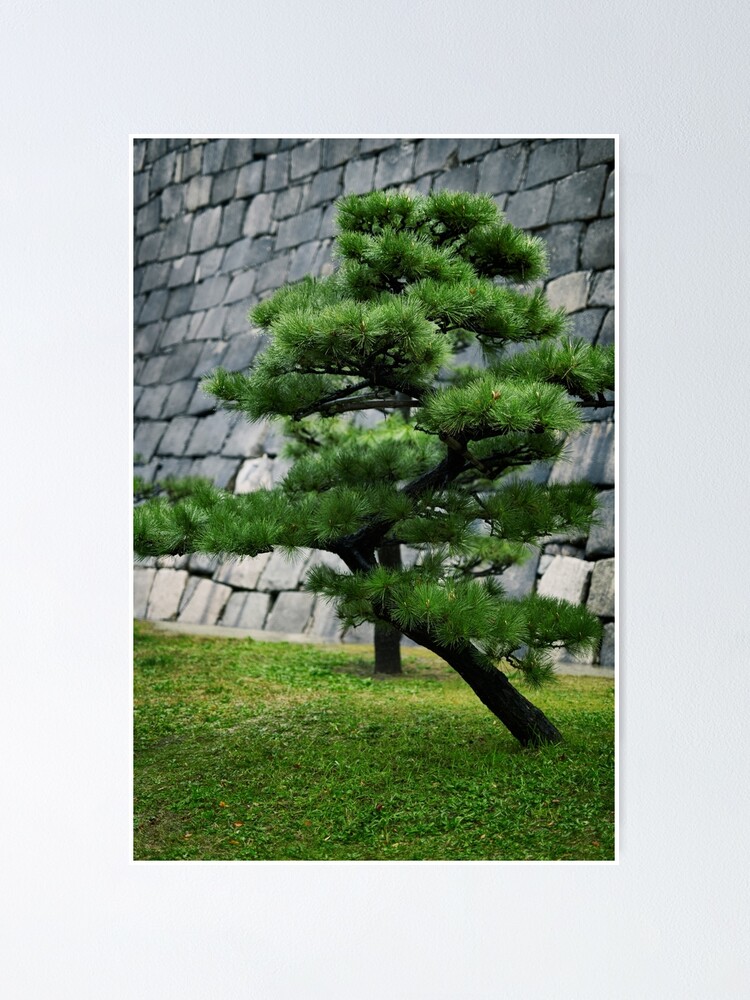This photograph captures an outdoor scene featuring two distinctive trees and a prominent stone wall. The tree closest to the viewer, situated at the bottom right, has a uniquely tilted trunk that curves upwards in a manner reminiscent of a bonsai, suggesting it's possibly a juniper with green, needle-like leaves. Directly behind it is a second tree that grows more straight up but is partially obscured by the front tree. Both trees are rooted in a well-maintained, short grassy lawn. The background is dominated by a massive stone wall composed of mostly dark grey stones, accented with a few lighter grey ones. This wall extends much higher than the visible trees, and its top is not visible within the image, hinting at its impressive height. The whole image is bordered by a light grey, thin frame, giving it a finished, print-like appearance with subtle textures noticeable in the upper right corner. The overall setup creates a serene, well-composed outdoor vista.